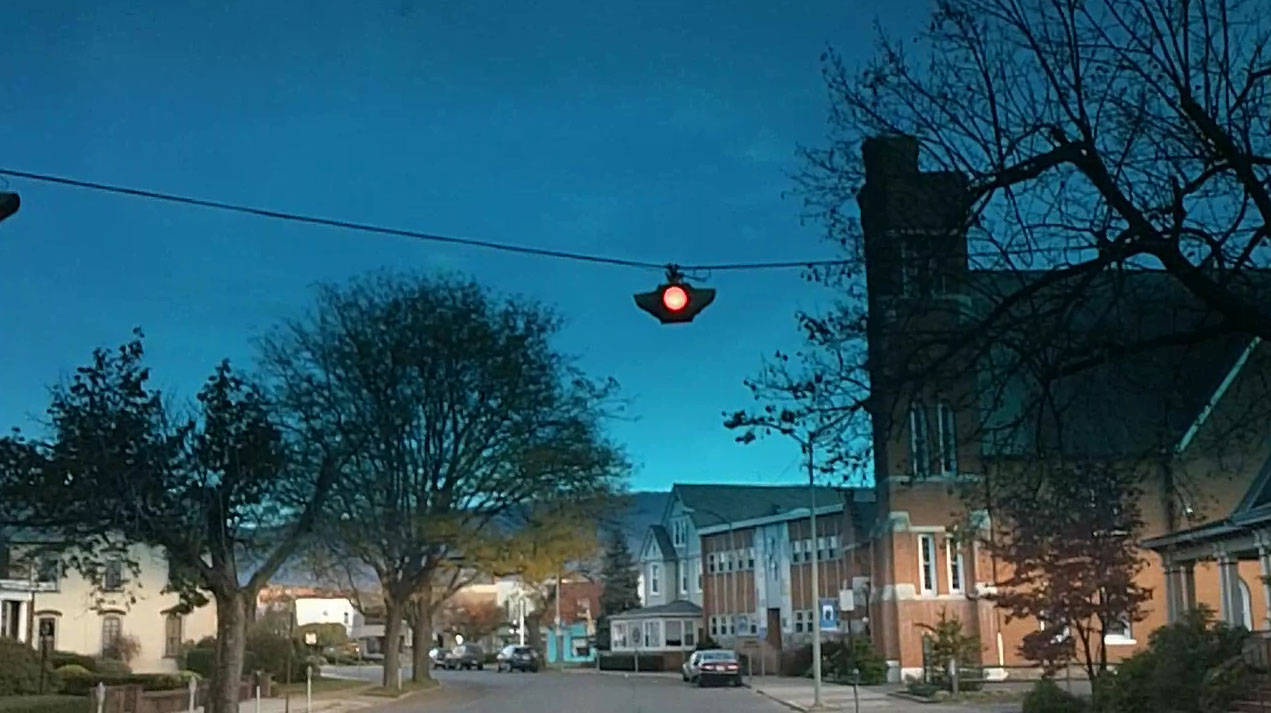This detailed color photograph captures a tranquil scene in a small suburban area in North America. The snapshot, taken from a first-person perspective, possibly from within a car, features a horizontal and rectangular composition. The viewer's attention is immediately drawn to a single yellow traffic light hanging from a wire that transsects the entire image. This light, appearing to direct traffic from all directions, suggests an intersection.

To the right of the street, a series of buildings with varying architectural styles stretch away from the camera. A series of brick buildings, followed by a wooden structure, and finally a small light blue building add character to the scene. On the left side of the street, a beige house stands quietly, accompanied by a sidewalk and deciduous trees, hinting at a temperate North American climate.

The sky is vibrant and blue, dotted with sparse clouds, suggesting the time is either early morning soon after sunrise or late in the day approaching dusk. The peaceful nature of the scene is emphasized by the few cars parked along the right-hand curb and the quiet residential feel. In the lower right-hand corner, part of a house porch and some bushes frame the scene, complemented by a small maple tree in front. This image captures the serene essence of suburban life, marked by its calm streets and modest architectural details.